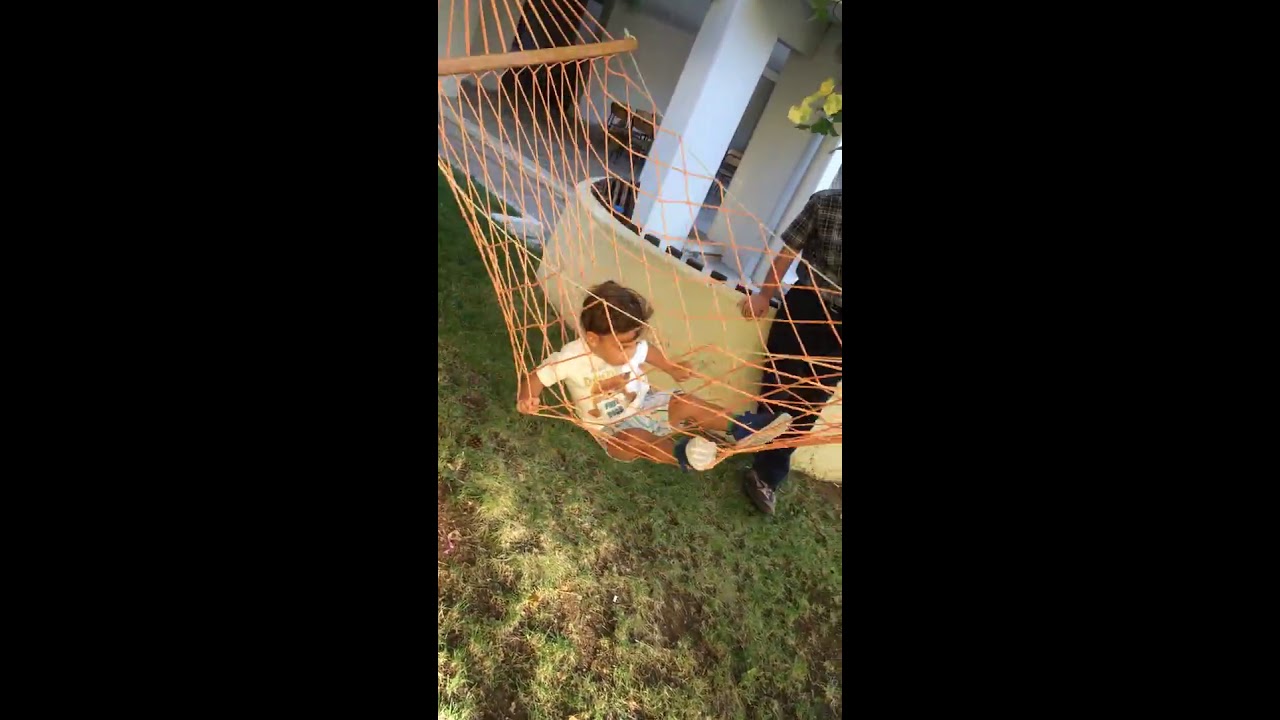In this detailed image set in a backyard, a toddler is relaxing in a large orange string hammock, which hangs over green grass speckled with patches of brown earth. The child, who appears to be of Hispanic descent with darker skin, is dressed in a white t-shirt and blue striped pants, complemented by blue shoes. The t-shirt features a design or lettering, though it is too blurry to decipher. 

An adult, also included in the scene, stands in the background wearing a plaid short-sleeve shirt and black pants. The adult's face is not visible, but one of their hands can be seen resting on a circular wall near a white house, which appears in the upper right of the image at an angle. Behind the adult, a porch with columns and a floor is partly visible, along with a tree adorned with yellow flowers and green leaves. The setting is illuminated by sunshine, creating a warm, inviting atmosphere.